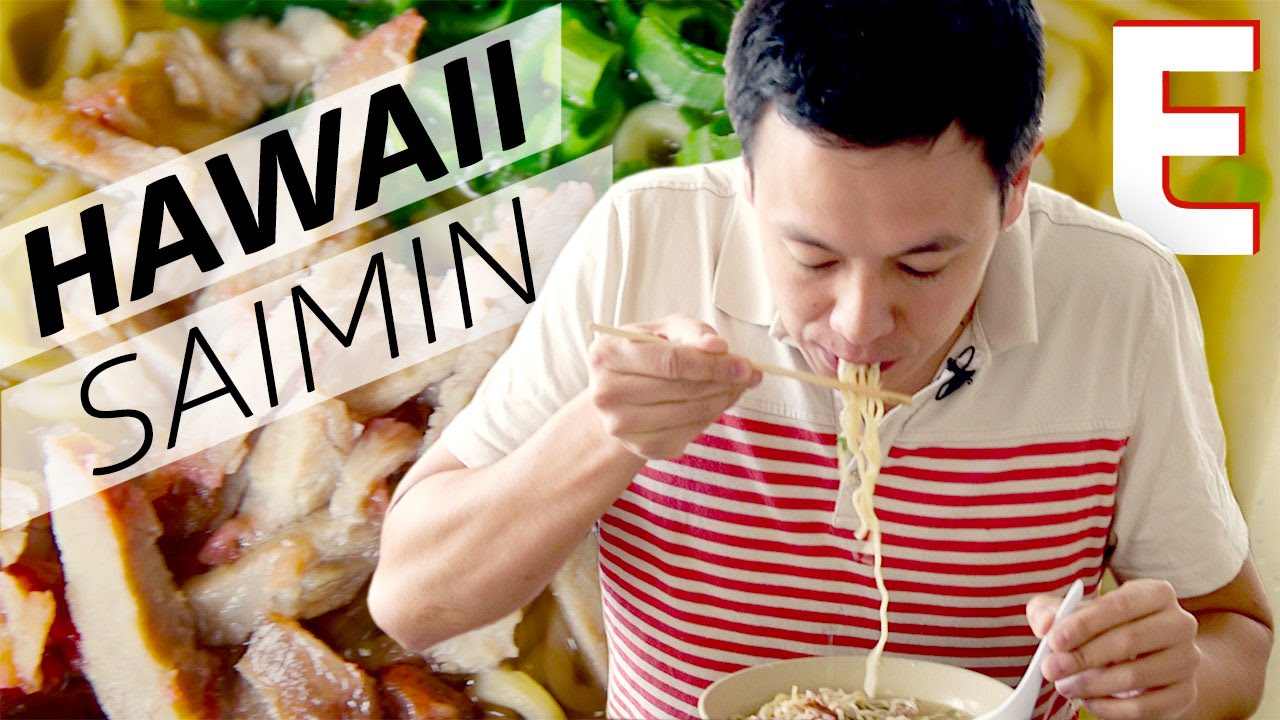In the advertisement, a young man in a short-sleeved, white collared shirt with horizontal red stripes is depicted eating noodles. Using chopsticks in his right hand and a white spoon in his left, he has a mouthful of noodles. Above him in big black capital letters, it reads "Hawaii Saimin." Measuring the same orange-pink hue that outlines a giant white letter 'E' on the left side of the poster, the stripes on his shirt add a cohesive color scheme. In the background, an image features slices of chicken and chopped green onions, likely ingredients in the noodle dish, enhancing the overall appeal of the meal being advertised. A microphone near his mouth suggests a demonstration or commentary, and the setup visually emphasizes the savory, hearty nature of the dish he's enjoying.